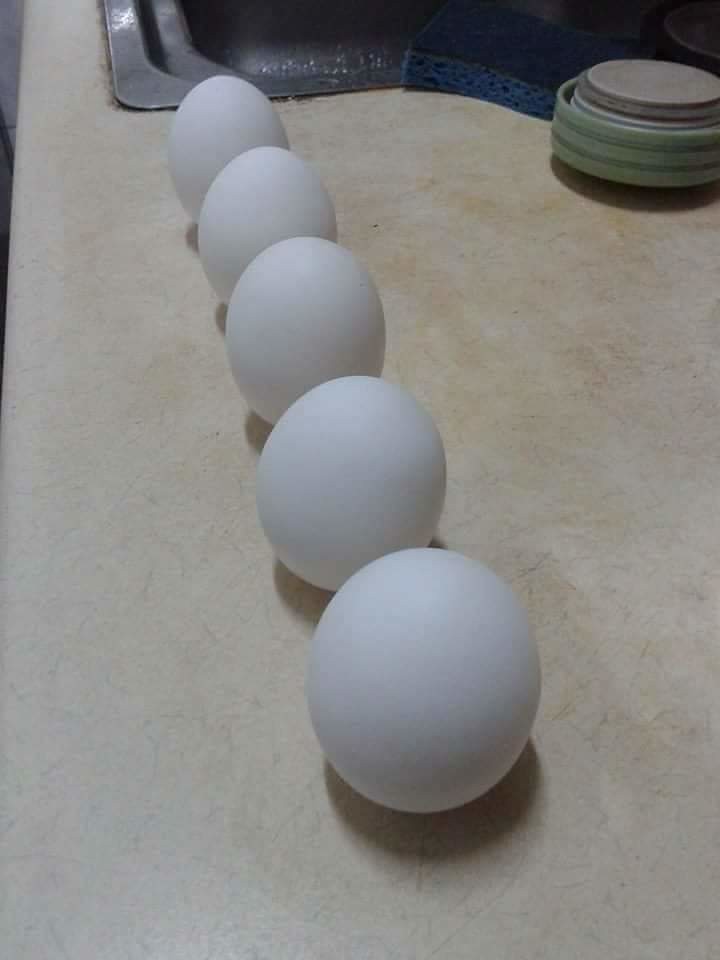A detailed photographic image captures five white eggs standing vertically on their ends in a diagonal line. The eggs are placed side by side on a light-colored countertop with a slight gray marbling effect. The image, taken from slightly above, creates a perspective that makes the eggs appear to stretch diagonally into the distance from the lower left to the upper right. The surface beneath them resembles a worn, yellowish-white Formica, with visible dark orange spots marking signs of age. In the background, an upside-down thermos lid sits in the back corner. Additionally, a gray metal tin, a blue scrubby sponge, and a green pottery bowl with dark green stripes containing an indistinct item are also visible to the right. The kitchen sink, with some dirt around the edges, adds to the composition of this everyday kitchen scene.